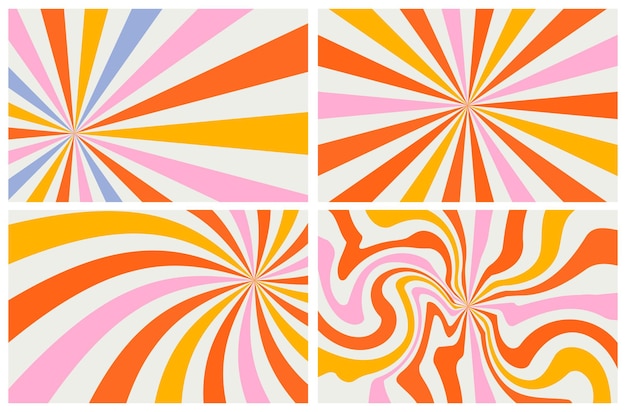The image depicts four equal-sized rectangular panels, each framed by a white cross-shaped divider. These panels exhibit intricate, psychedelic designs reminiscent of the 1960s, featuring vibrant rays emanating from a central point. The color scheme predominantly includes dark orange, light orange, and pink, with the top left panel distinctly incorporating shades of blue. 

The top left panel's rays converge towards a point slightly offset from the center, giving it a unique asymmetrical look. The top right panel displays more uniformly centered radiating orange, yellow, and pink lines. At the bottom left, the design shifts with curved lines emanating from a point in the top right corner, suggesting a gentle twist in the rays' formation. Lastly, the bottom right panel features very wavy and squiggly lines radiating from a central point, adding a further layer of dynamic, almost contorted motion to the overall composition.